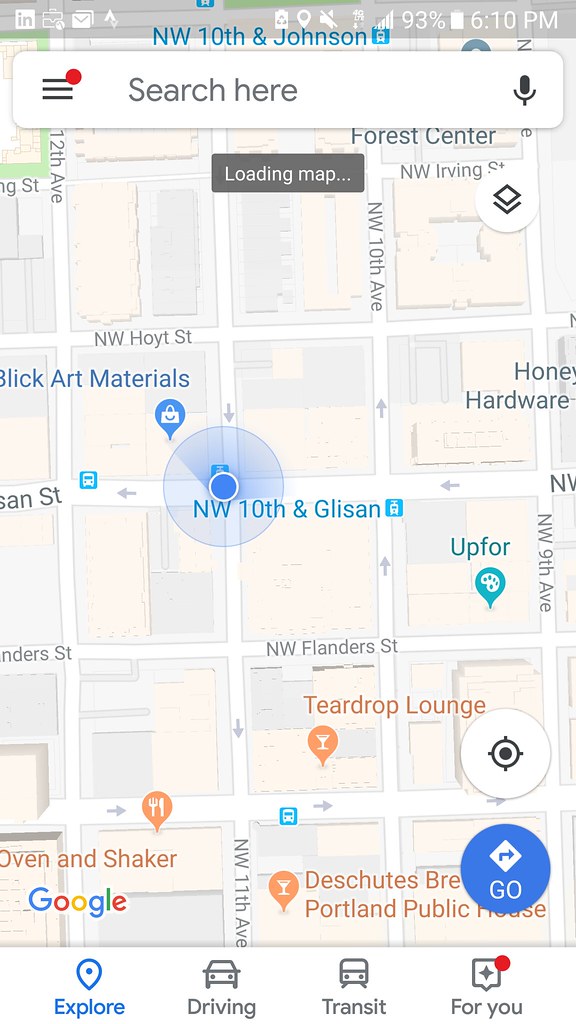This image is a detailed screenshot from a mobile device displaying a Google Maps interface. At the top of the screen, a gray status bar includes various white icons such as LinkedIn, Gmail, a paper plane, battery level indicator, location pin, a muted speaker, the battery percentage (93%), and the time (6:10 p.m.).

Below the status bar, the Google Maps interface is shown. A white search box at the top contains the text "Search here" alongside a black microphone icon. The map itself features various gray lines and a prominent red dot, indicating a specific location. The view appears to be in a street view mode, with a color scheme that includes shades of tan, gray, blue, orange, and white. A gray box with the text "Loading map" is visible on the screen.

The map labels several landmarks and streets, including Forest Center, Northwest Irving Street, Northwest 10th Avenue, Northwest Hoyt Street, Blink Art Materials, Northwest 10th and Glisan, Upthor, Honey Hardware, Northwest Flanders Street, Teardrop Lounge, Oven and Shaker, and Portland Public (with the rest of the text cut off). 

A prominent blue circle with white text reading "Go" is also displayed. At the bottom of the screen, a blue location pin icon indicates the "Explore" tab. Next to this are icons and labels for other navigation options: "Driving" with a gray car icon, "Transit" with a bus icon, "For you" with a banner and star icon, and a red dot. Above the "Explore" tab is the recognizable Google logo.